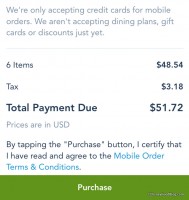A cropped screenshot from a mobile order for a Disney quick service restaurant. The background is predominantly white, with a green bar at the bottom displaying the word "Purchase." At the top, a message informs users that only credit cards are accepted for mobile orders—no gift cards, dining plans, or discounts are currently allowed. 

Just below this notice, the details of the order are itemized: "6 items" are listed, totaling $48.54. Adjacent to this, "Tax" is specified at $3.18. The "Total Payment Due" is prominently displayed in large, bold black letters, amounting to $51.72, also in bold black numbers. Directly under this total, a note states that all prices are in USD.

Above the green purchase bar, there is a disclaimer in smaller text: "By tapping the purchase button, I certify that I have read and agreed to the mobile order terms and conditions." The phrase "Mobile Order Terms and Conditions" is in blue, indicating it's hyperlinked and can be clicked to view further details. All other contextual information outside of this described section is cropped out from the screenshot.